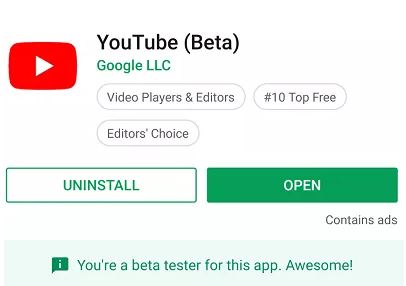A screenshot from the App Store displaying the YouTube Beta app by Google LLC. The app is categorized under "Video Players & Editors" and is listed as number 10 in the top free apps, also marked with an "Editor's Choice" label. The interface shows two buttons: "Uninstall" (with a white background and green text) and "Open" (with a green background and white text). There is also a note indicating that the user is a beta tester for this application, along with a notice that the app contains ads. The slightly dated YouTube logo suggests this screenshot is from an older version of the app when it was still in its beta testing phase, before becoming the ubiquitous platform it is today.